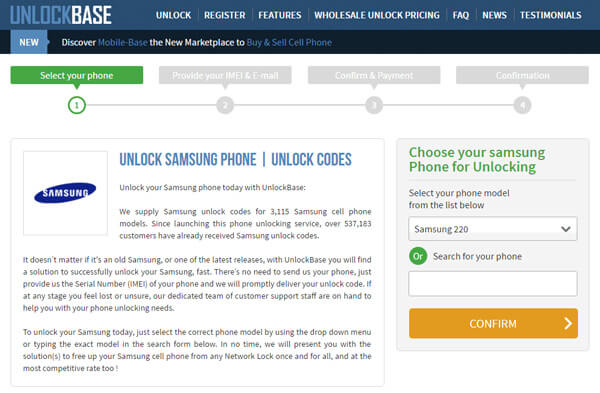This detailed caption goes with the screenshot of the Unlock Base website:

---

The screenshot captures the website interface of Unlock Base, showcasing its navigational and functional features. At the top, the navigation menu includes options such as "Unlock," "Register," "Features," "Wholesale Unlock Pricing," "FAQ," "News," and "Testimonials." Beneath this menu, highlighted in a light blue box, it announces "Discover Mobile Base" - a new marketplace for buying and selling cell phones.

The main content area features a streamlined, step-by-step unlocking process for mobile devices, starting with "Select Your Phone," highlighted in a green box as the first active step. Following this, subsequent steps "Provide Your IMEI and Email," "Confirm and Payment," and "Confirmation" are grayed out, indicating they will activate sequentially.

Below this process guide, the website highlights specific services for unlocking Samsung phones. Accompanied by the Samsung logo, the text promotes their Samsung Unlock Codes, applicable to 3,115 Samsung models. A significant milestone is emphasized: over 537,183 customers have successfully received Samsung Unlock Codes since the service's inception. The text reassures users of a straightforward, device-independent solution requiring only the phone's serial number (IMEI). Customer support is available to assist at any stage of the process, ensuring a smooth experience.

To initiate the unlocking process for a Samsung phone, users are instructed to select their specific model from a dropdown menu or search for it by typing in the search form provided. This section concludes with an orange "Confirm" button, guiding the user to finalize their selection and proceed with unlocking their device.

---